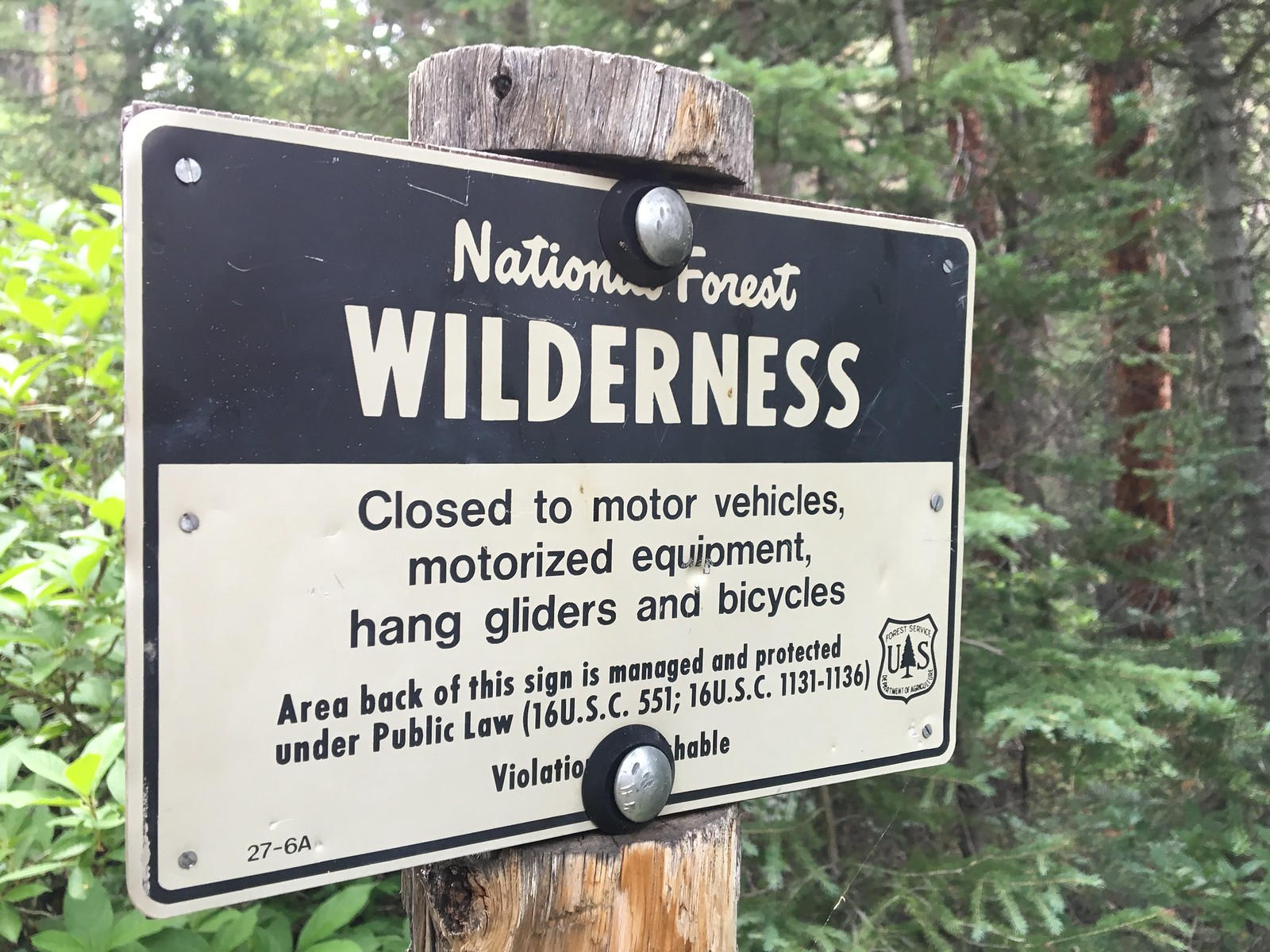This color photograph, taken on a sunny day in a forest, captures a metal sign bolted to a sturdy wooden post. The sign reads: "National Forest Wilderness. Closed to motor vehicles, motorized equipment, hang gliders, and bicycles. The area beyond this sign is managed and protected under public law 16 U.S.C. 55, 16 U.S.C. 1131-1136 by the United States Department of Agriculture. Violations are punishable." The vibrant greenery of the forest and clear blue sky add a serene backdrop to the image, emphasizing the importance of preserving this natural area.